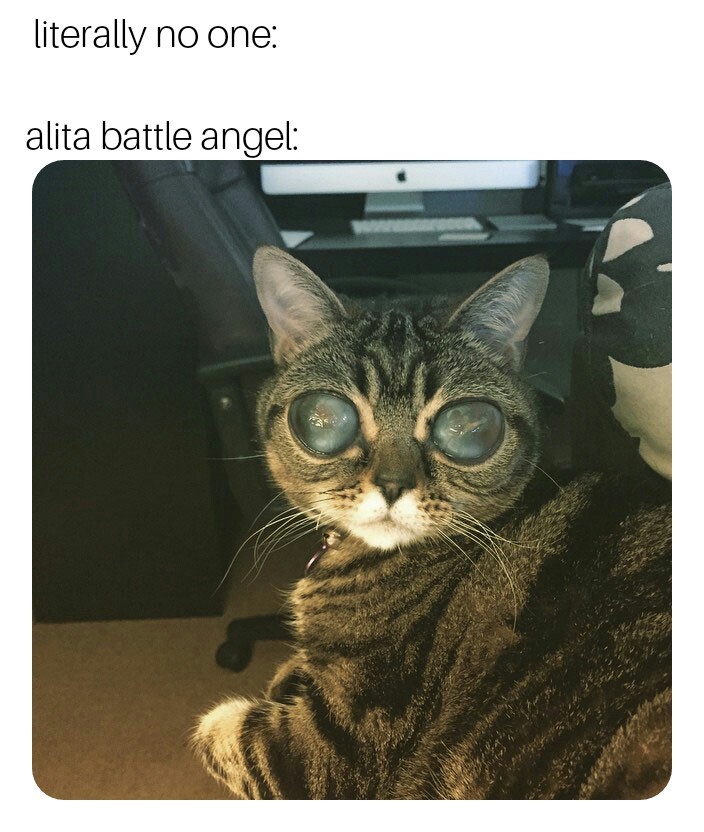The image is a humorous meme featuring a close-up photo of a small calico cat with uniquely large, circular eyes resembling those from a Margaret Thiem painting or a Snapchat/Instagram filter. The cat, which has white whiskers, white paws, and a small, pointed nose and mouth, is lying down but looking back towards the camera with cloudy green eyes, making it appear almost like a kitten. The cat is situated in an office-like setting; visible behind it is the bottom part of a Mac computer monitor, a silver keyboard, and a black desk chair. At the top of the image, black text reads "literally no one:" followed by a colon. Below that, another line of text says "Alita Battle Angel:" introducing the comical depiction of the cat with its exaggerated, anime-like eyes.